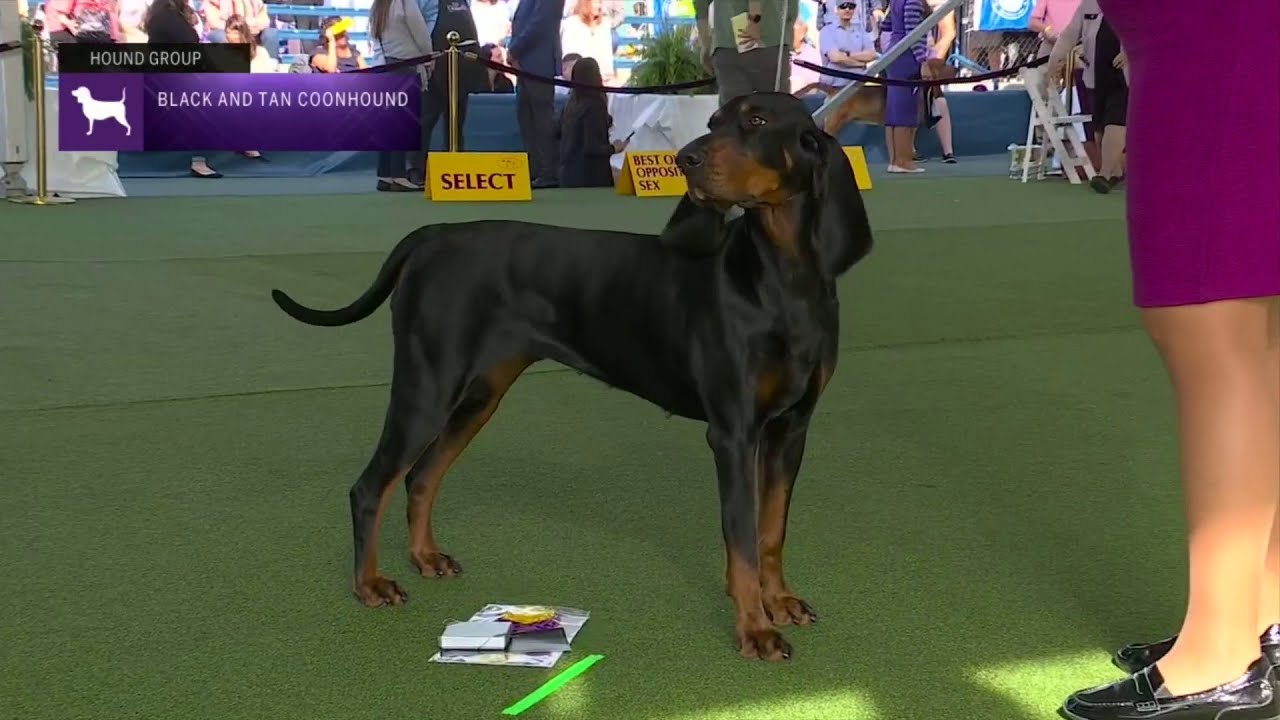The photo captures a dog show, featuring a Black and Tan Coonhound prominently displayed at the center. The dog's body is mostly black with distinctive brown markings on its feet, snout, and neck. It has long, floppy, non-cropped ears and a long, skinny, non-cropped tail. The dog stands on green, indoor-outdoor type carpeting, typical of artificial turf grass, and is looking to the left. A woman, partially visible, is holding the dog on a leash. She is dressed in a burgundy or wine-colored skirt and black loafers. To the left, near the bleachers, there's a purple sign with a white silhouette of a dog and text reading "Black and Tan Coonhound." The scene includes some papers and documents in the foreground, likely related to the competition, and faintly visible people in the background near the seats. The photo hints at a professional setting, possibly even televised, as suggested by the overlay in the upper left corner indicating "Hound Group" and featuring the "Black and Tan Coonhound."